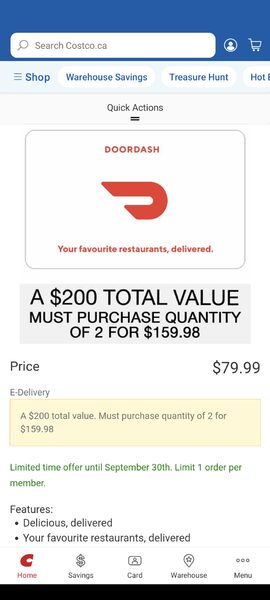The image appears to be a screenshot from a website, most likely DoorDash, as indicated by the logo featured on the webpage. The webpage prominently displays Costco CA at the top, suggesting that this page relates to shopping at Costco via DoorDash. There is a search bar, followed by categories such as "Shop," "Warehouse Savings," and "Treasure Hunts."

An advertisement occupies a significant portion of the page, mentioning, "Your Favorite Restaurants Delivered." Just below this, there is a detailed offer: "Total $200 value must purchase quantity of two for $159.98." This implies that the user has a $200 total value deal, but it must be purchased in quantities of two, each priced at $79.99. This offer highlights that it's an "E-Delivery."

The offer reiterates in green text, "Limited-Time Offer until September 30th, limit one order per member." Features mentioned include "Delicious Delivered" and "Your Favorite Restaurants Delivered."

At the very bottom of the screenshot, there are a series of icons, each representing different sections: a red 'C' for Home, a gray dollar sign for Savings, a gray card for Cart, a gray image icon for Warehouse, and a menu icon with three dots above it. Notably, the top of the page lacks any clear branding from a specific store or company name.